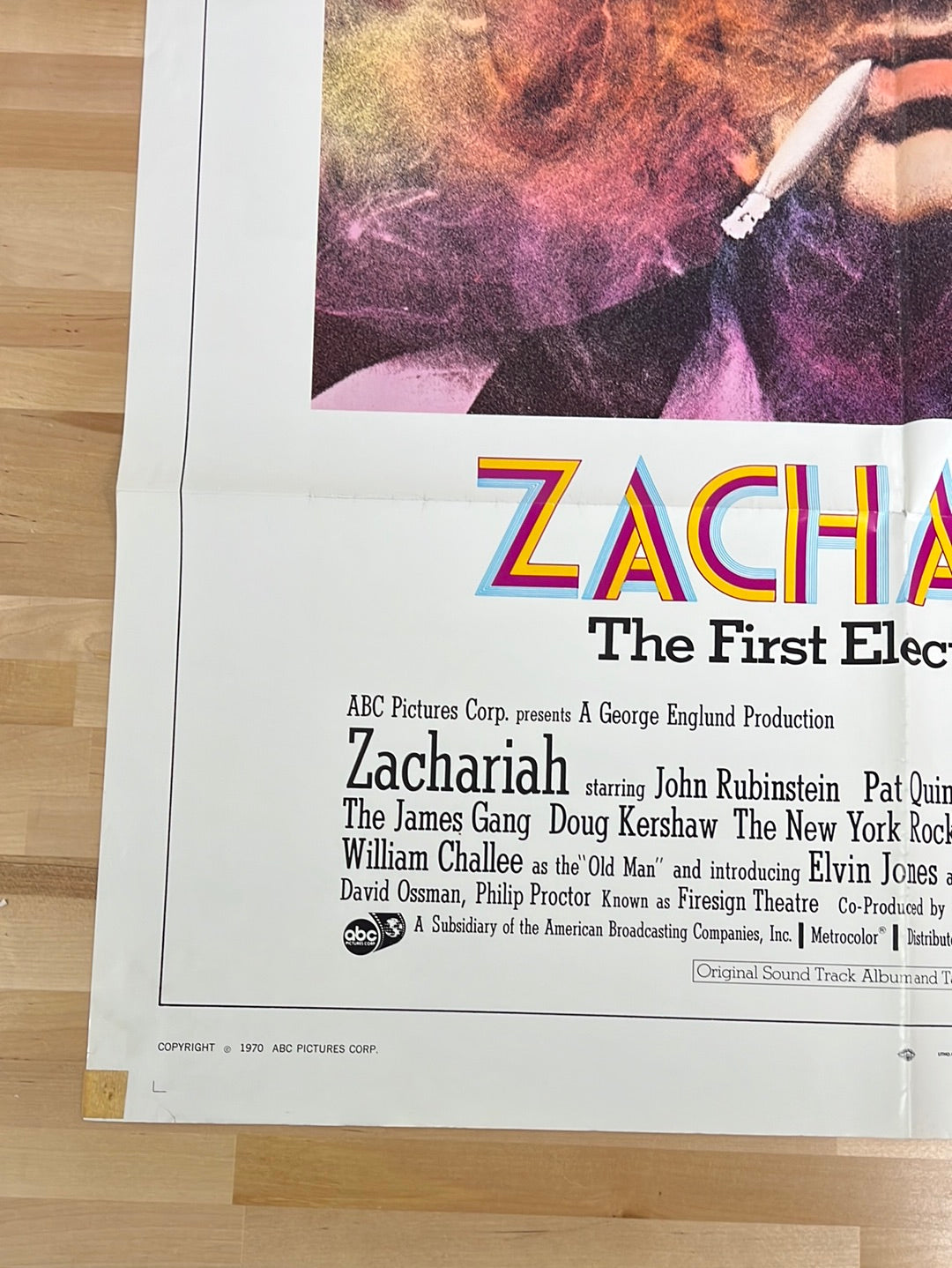The image depicts a partially cropped poster laid on a light, hardwood floor, with a piece of brownish tape affixed to the bottom left corner. The primary focus of the poster is the bold text "Zachariah" prominently displayed in vibrant yellow, magenta, and blue letters. Despite some cropping, the following details are visible:

- At the top right, there's a photo, possibly of a man or woman, with partially visible facial features, including pink lips, white skin, and a cigarette emitting purple-toned smoke obscuring the upper part of the face.
- Below the photograph, the text "Z-A-C-H-A" appears in the same colorful letters.
- The words “the first ELEC” are partially visible, with the rest obscured.
- Additional text reads, "ABC Pictures Corp. presents a George England production, Zachariah starring John Rubenstein, Pat Quinn, the James Gang, Doug Kershaw, the New York Rock, William Chalee as the old man, and introducing Elvin Jones, David Osman, and Philip Proctor, known as Firesign Theater."

The poster is co-produced by a subsidiary of the American Broadcasting Companies Incorporated and showcases the use of MetroColor. An original soundtrack album is mentioned. A black border frames the bottom and part of the left side of the poster. At the bottom left corner, the text "Copyright 1970 ABC Pictures Corp." is clearly visible.